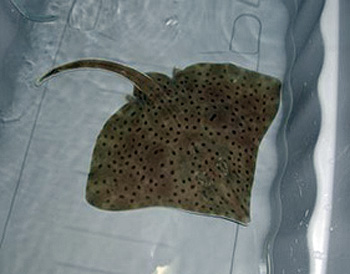This photograph captures a small stingray in a shallow, bright white plastic container, likely used in an aquarium setting. The container is filled with just a few inches of water, enough to keep the stingray submerged and alive. The stingray, predominantly a mottled brown and green with various shades of brown, features an array of black spots across its body, giving it a camouflaged appearance. With eyes positioned on top of its long, triangular body and a long, dangerous tail extending upwards and to the left, the stingray displays the characteristic markings and structure of its species. The naturalistic lighting enhances the texture of the water, revealing small ripples and reflections. The stingray's tail, known for storing poison, gently touches the wall of the container, highlighting the creature’s confinement within the small pool.